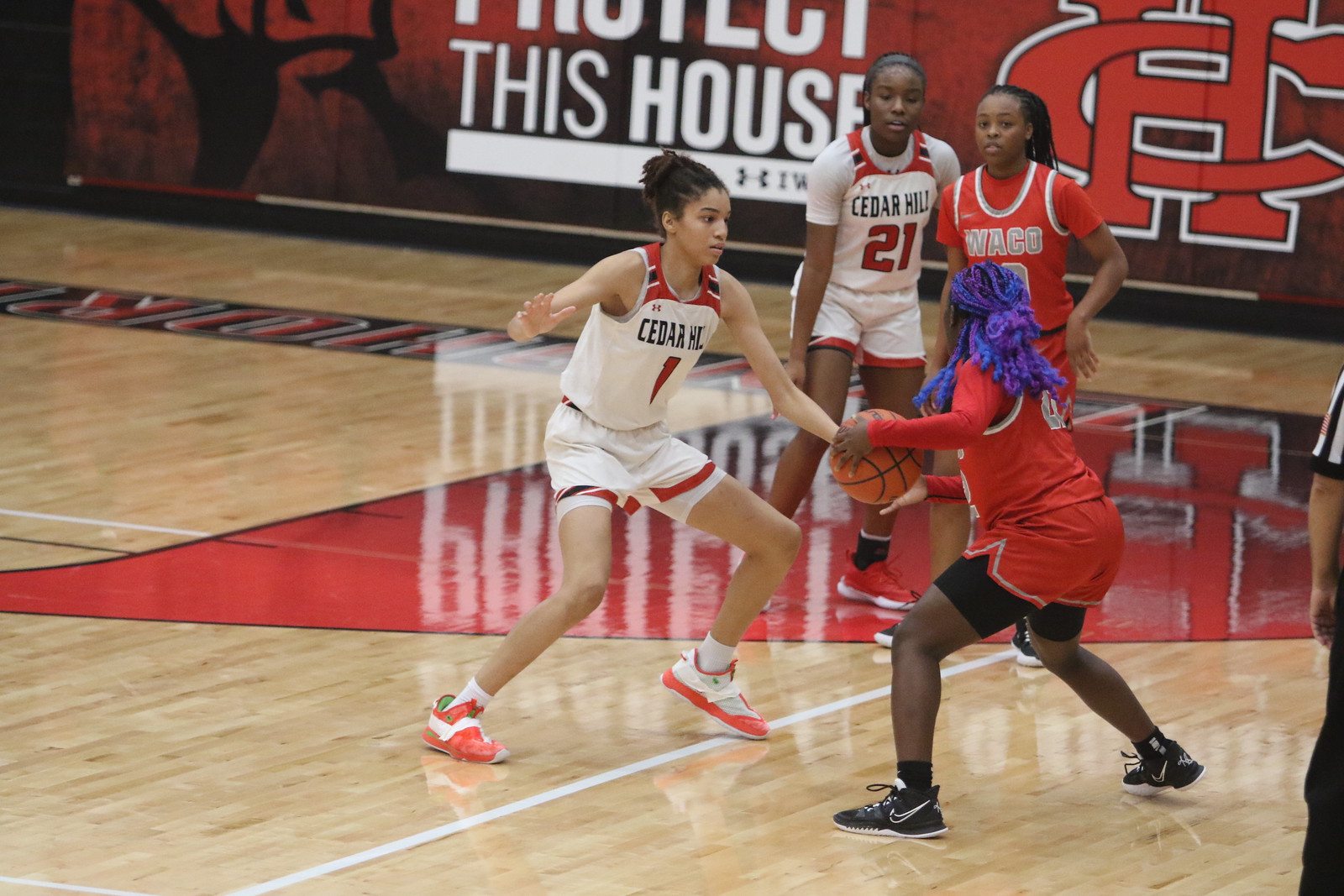The image depicts a high school girls' basketball game on a shiny, brown wooden court. In the foreground, a girl with purple hair tied back wearing a red uniform with black shorts and black sneakers is holding the basketball. She appears to be guarded by a girl in a white jersey with red and blue accents that reads "Cedar Hill," who is wearing white shorts with red trim and red sneakers. Another player from Cedar Hill, with her hair also pulled back, is visible next to her, sporting the number 21 on her white uniform with matching shorts. Both Cedar Hill players have a red, white, and blue stripe on their shoulders. Off to the side, in the lower part of the image, an arm and part of a leg of a referee in a black and white striped shirt and black pants are visible. The background showcases a wall with advertisements, and prominently features a red and black team logo with the intertwined letters "CH" along with the phrase "This House."